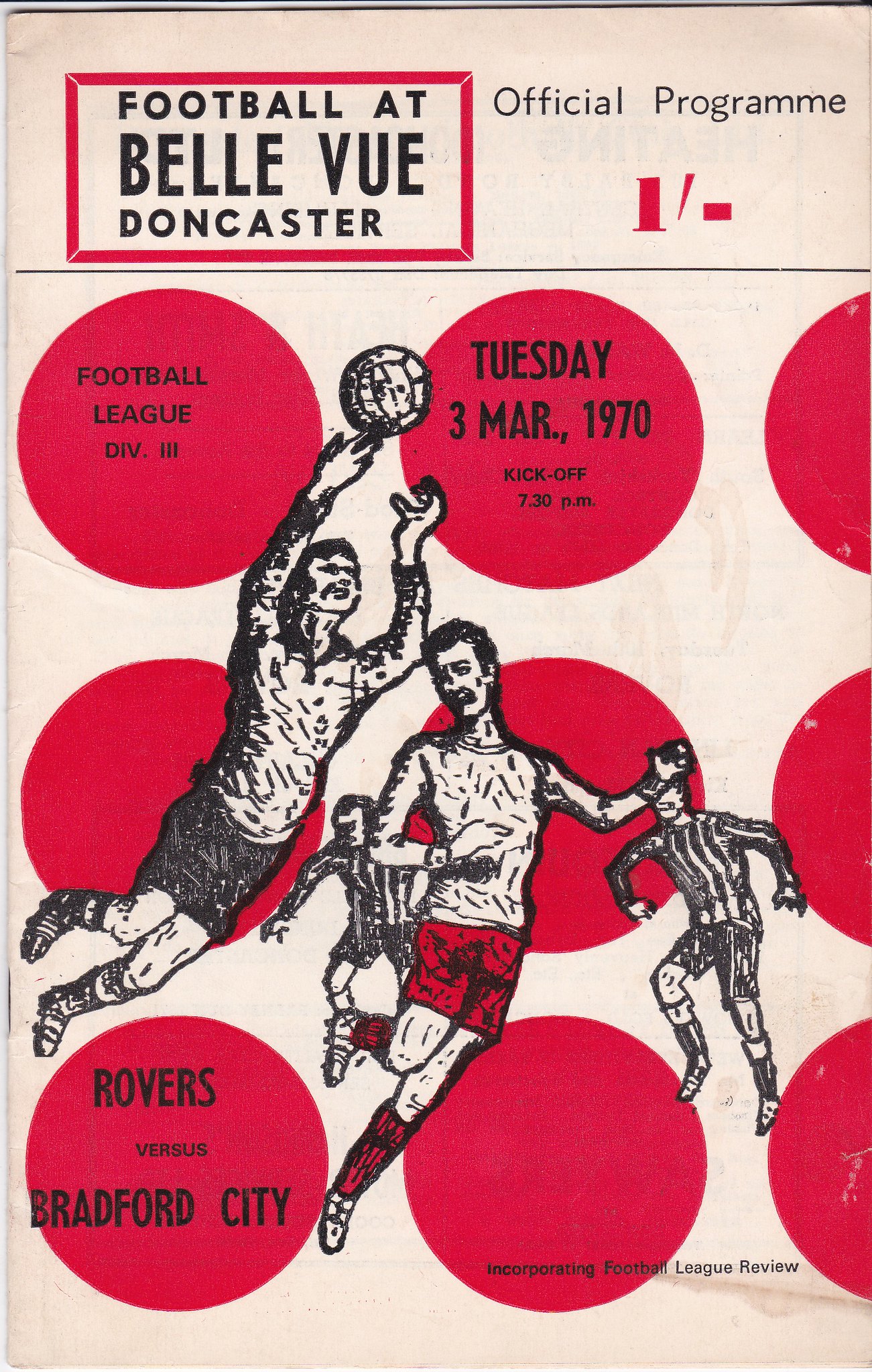The cover of this vintage football program features a slightly aged white background with a narrow red rectangular outline at the top. Inside the rectangle, bold black text reads "Football at Bellevue, Doncaster," followed by the words "Official Program" and a large number "1." To the left, a smaller circle in black text details the event as "Football League Division Three," with "Tuesday 3 March 1970, Kickoff 7.30 p.m." prominently displayed. Below this, there are about nine large solid red circles, though three on the right are cut off, making them appear as half circles. The bottom left circle is inscribed in black with "Rovers vs. Bradford City," while the others remain blank. A central illustration depicts two soccer players in light-colored shirts, with one wearing black shorts and the other in red, both leaping for a soccer ball. In the background, two referees watch, ready to take positions once the ball descends. The bottom right corner notes "Incorporating Football League Review." The layout exudes a nostalgic charm, reflective of a bygone era in football history.